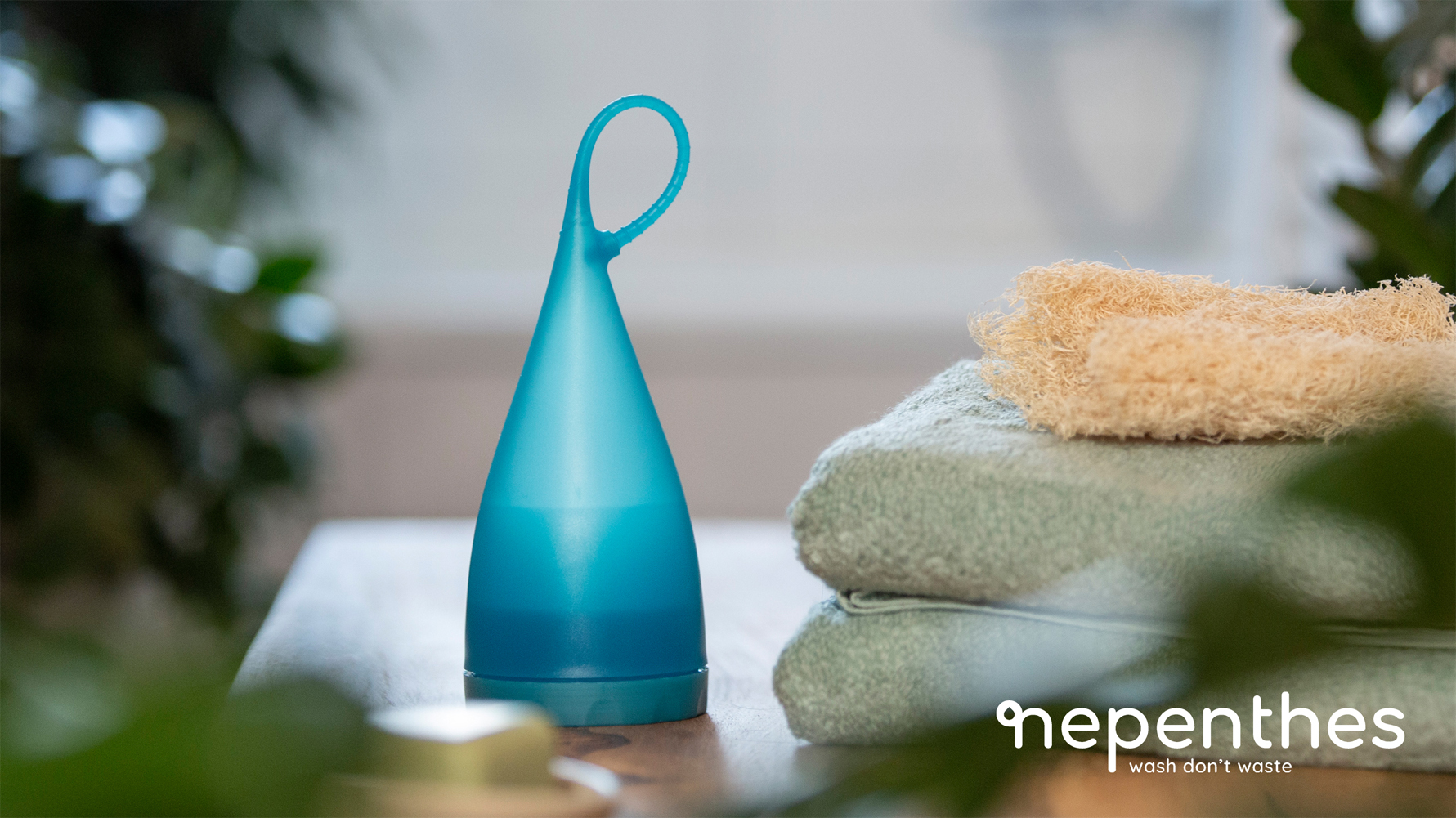This image, likely an advertisement, captures a serene, spa-like bathroom setting. The focus is on a wooden countertop in the foreground, where two neatly folded, light green towels lie next to a cream-colored loofah. To the left of the towels is a light blue, teardrop-shaped device with a loop at the top, reminiscent of a menstrual cup. The background features a heavily blurred bathtub, some dangling coils, and various plants, contributing to the calming ambiance. In the bottom right corner, the text "Nepenthes Wash Don't Waste" is prominently displayed in white font.